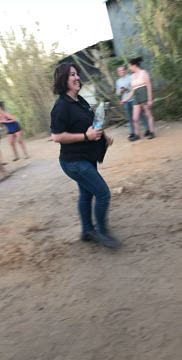In this outdoor photograph, a woman is captured mid-stride in the foreground, her movement rendering her feet slightly blurry as one lifts off the sandy ground. She is dressed in tight-fitting dark blue jeans paired with dark shoes and a short-sleeve black blouse adorned with a collar. Accessorizing her look, she sports a black watch on her wrist and carries a clear plastic water bottle. Her shoulder-length dark brown hair frames a beaming smile.

In the background, two individuals, a man and a woman, stand closely together, sharing smiles and an evident moment of connection. To their left, partially visible, is the body of another young woman. She is bent over with her knees bent, seemingly engaged in a gesture directed toward someone out of frame.

The scene is set against a backdrop featuring a gray stone building and tall, dry bushes, adding a rustic ambiance to the photograph.